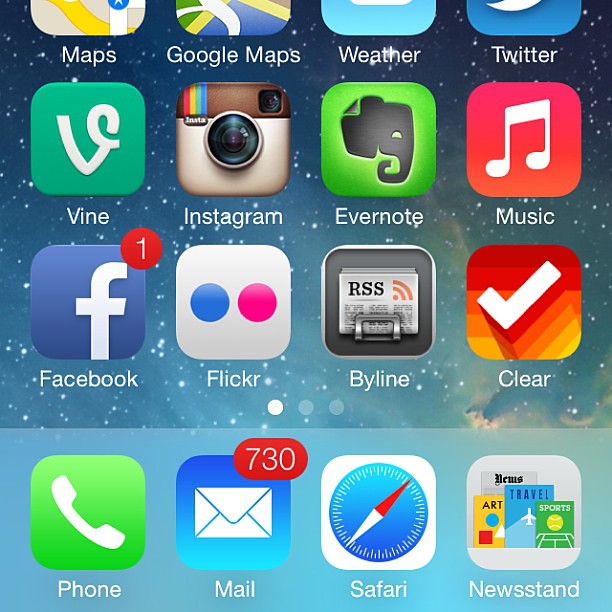The image displays a vibrant and colorful smartphone home screen, brimming with an array of different apps. From the top, starting on the left, there are icons for Maps, Google Maps, Weather, and Twitter. Below these, the next row includes apps for Vine, Instagram, Evernote, and a generic Music app. Facebook is also present, signified with a notification badge showing one alert.

Continuing down, the next section houses icons for Flickr, Byline, Clear—with its prominent white check mark—Phone, Mail (displaying 730 unread messages), Safari, and Newsstand. The Newsstand app showcases a variety of miniature magazine covers, encompassing themes like Art, Travel, Esports, and News.

The entire home screen is set against a light blue background peppered with white dots, augmenting the overall kaleidoscope of vivid hues. The app icons themselves cover nearly the full spectrum of colors, including blues, teals, browns, yellows, golds, whites, blacks, various shades of blue, and pink. Each app stands out distinctly with its unique color scheme, creating a lively and engaging visual experience.